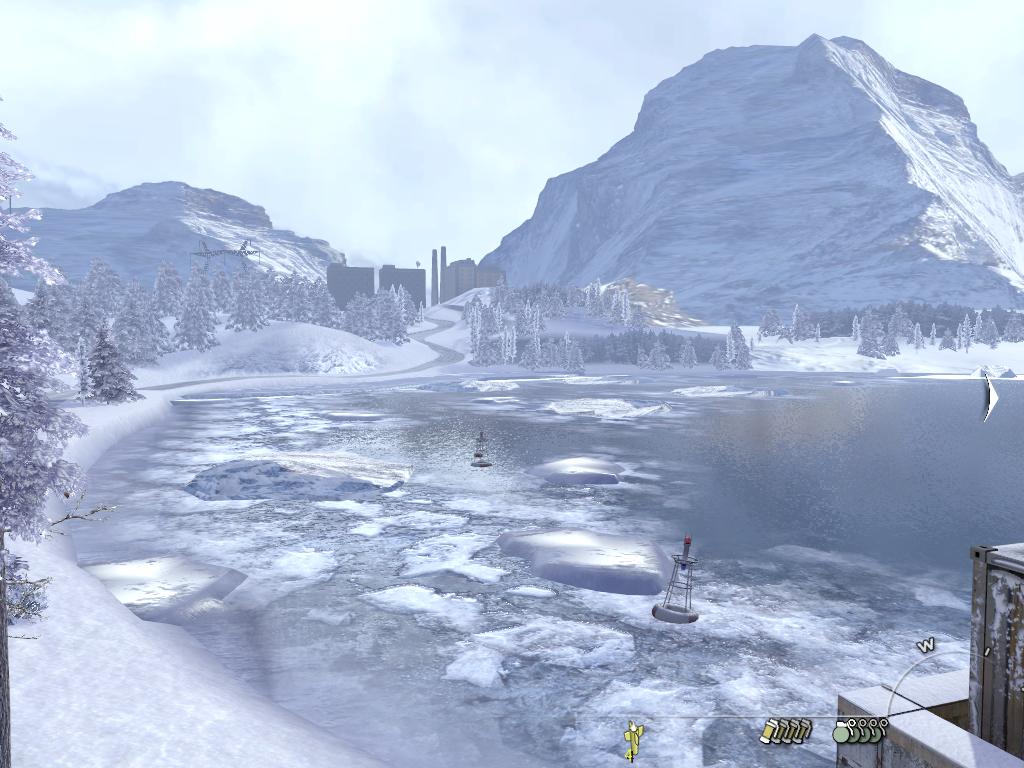This detailed caption combines elements from all three descriptions:

This image is a highly detailed screenshot from a modern 3D video game set in a bleak, icy environment reminiscent of Skyrim but with more contemporary elements. In the foreground is a mostly frozen lake adorned with ice blocks and two buoys—one caught in the ice and another slightly further away. The lake stretches towards the horizon, bordered by snow-covered evergreen trees and mountainous terrain. On the right-hand side of the image stands a tall mountain, which is half the height of a shorter mountain on the left. Between these peaks lie three tall buildings and two tall smokestacks, set amid the rugged landscape.

A winding road, edged with snow-laden trees, descends from the right-side mountain, meandering through the scene. At the bottom right corner of the image, there's a partially visible building with lines extending from it, accompanied by four round yellow tags, four cylindrical tags, and a tag shaped like a plane. An arc with a 'W' overhead highlights this area, indicating the west direction.

In the background, a foggy, cloudy sky partially obscures a large gate or entrance to a fortress, hinting at a larger, inhabited area beyond the ice-bound scenery. The game's interface is visible at the bottom right, showing icons for various grenades, including flash and smoke grenades, and a compass pointing slightly west, underlining the video game's navigational aspect.